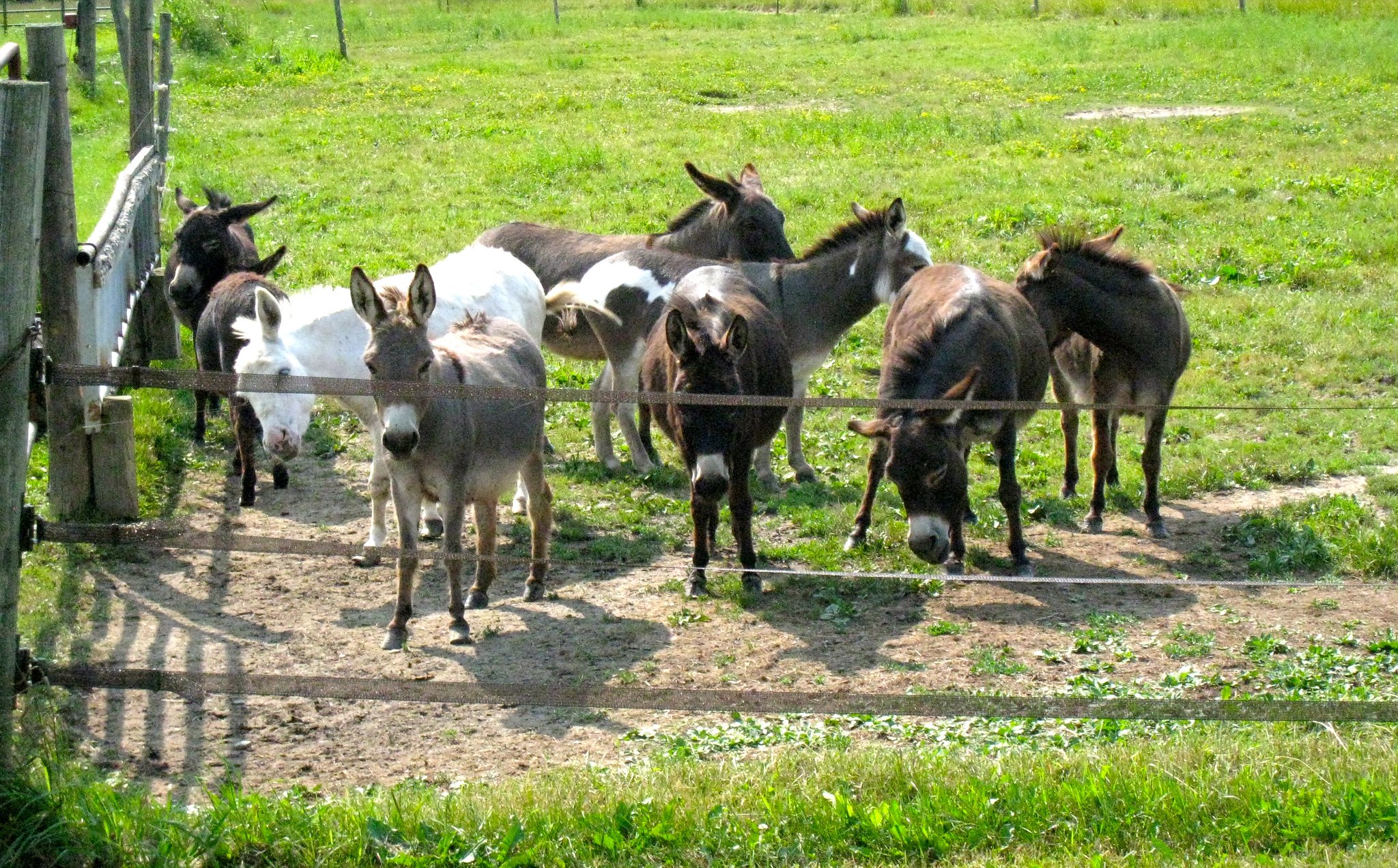This outdoor color photograph, taken in bright daylight, captures a group of approximately seven to eight burros, likely mixed with donkeys, within a corral. The corral is enclosed by electrified fabric tape fences and partially metal fences. Dominating the foreground are three burros facing directly towards the camera—a gray one on the left, and two brown ones on the right, with the furthest right burro having its head tilted down toward the ground. Among the variously colored burros in the image are a grayish brown, a reddish brown, a dark brown with white spots, a nearly black one, and a white one. Scattered throughout the background, we see more burros, including two gray and one white, all positioned with their heads turned to the right. The burros stand mostly on dirt, but the surrounding pasture area is lush with green grass, crisscrossed by well-trodden paths. The entire scene is free of any text or printing.